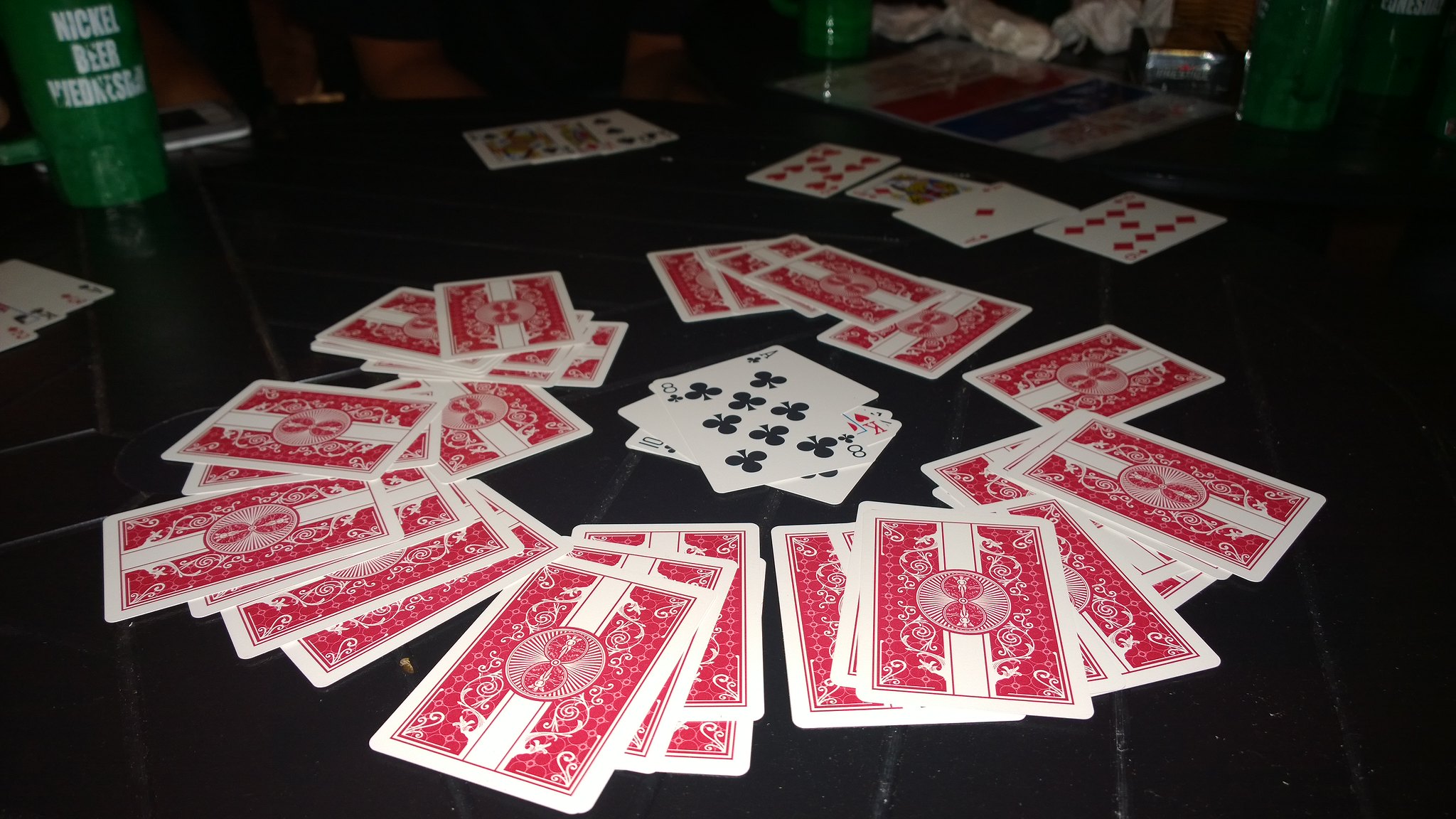The image captures an intimate indoor scene of a card game in progress on a wooden table. The deck features white and red backs, with cards laid out in somewhat untidy piles, suggesting the game is in mid-play. Among the scattered cards, visible face-up are an ace, a king, a queen, a jack, and prominently, an eight of clubs atop one of the seven piles. Each card pile is arranged face down, hinting at a structured game setup.

In the background, three players are participating, though their faces are not visible. Their cards are held openly, facing the center of the table, revealing approximately four cards each, indicating a game where hands are meant to be seen by all players. One player has a cup marked "knicker beer," albeit partially obscured by lighting.

Elements within the room add to the scene’s ambiance. A shiny, gray-silver object in the background, possibly a lighter or chrome accessory, catches some light, adding a hint of metallic gleam to the setting. This combination of specific details paints a vivid picture of a cozy game night among friends.